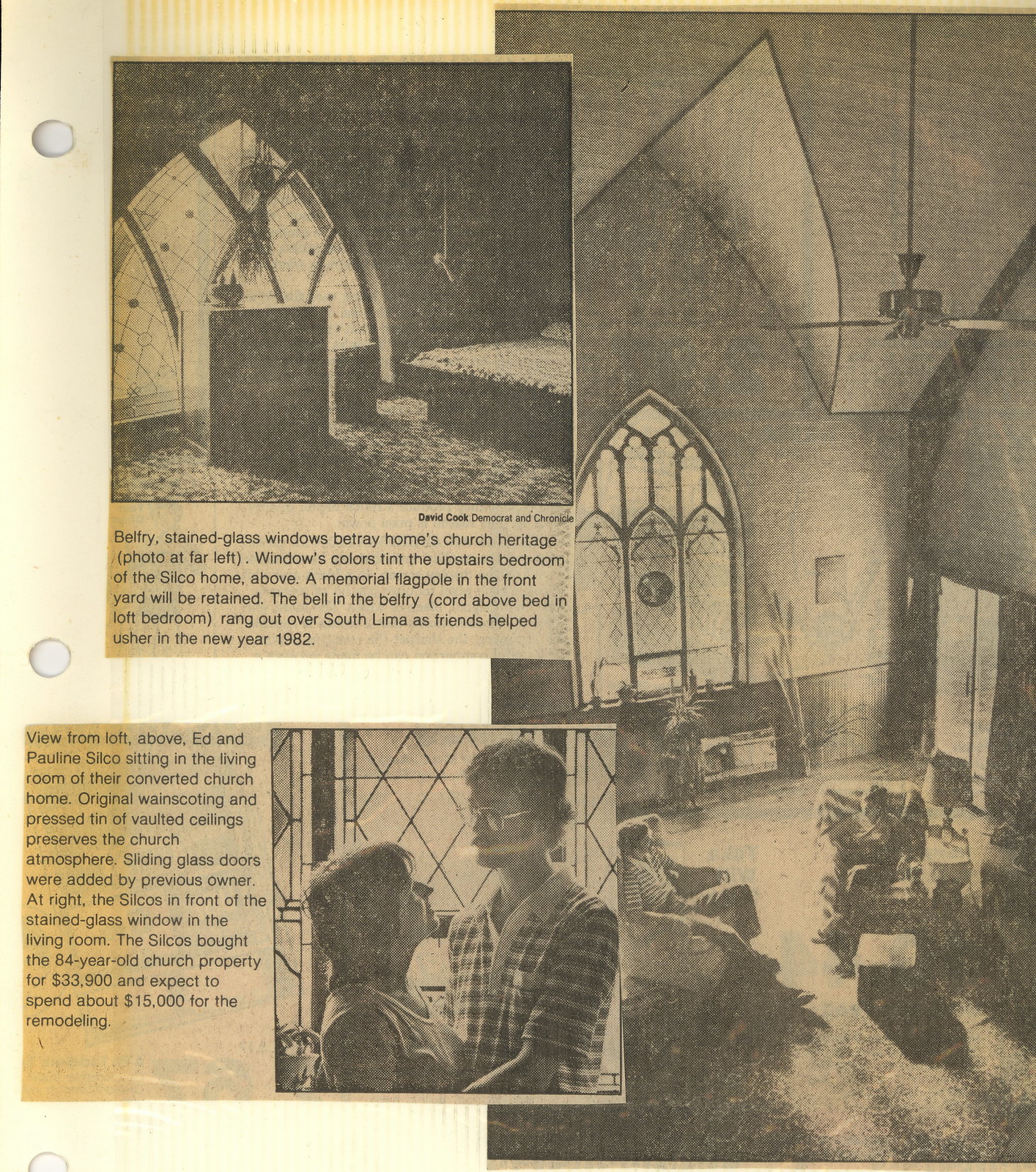The image depicts yellowed newspaper clippings preserved in a plastic sleeve with three punched holes on the left side, suggesting it belongs in a three-ring binder or photo album. The main feature of the clippings is a series of black-and-white photographs and articles detailing the transformation of an old 84-year-old church into a private home by Ed and Pauline Silco. 

There are three main photographs:

1. **Interior View of the Church**: Showcases the high vaulted ceilings with original wainscoting and pressed tin, emphasizing the preserved church atmosphere. The ceiling also has a ceiling fan, indicative of modern additions.

2. **Stained Glass Windows and Seating Arrangement**: Displays the intricate belfry stained glass windows, a key aesthetic element retained from the church, with a seating arrangement in front, highlighting how the church's heritage has been incorporated into the home's design.

3. **Ed and Pauline Silco**: The couple is seen in two settings—standing together in front of the stained glass windows, and sitting in their living room, demonstrating their personal connection to the converted church home. The article reveals they purchased the property for $33,900 and aimed to spend about $15,000 on remodeling.

Additional text on the clippings mentions that the stained glass windows cast colorful tints in the upstairs bedroom, and a memorial flagpole in the backyard will be retained. A bell in the belfry, located above the loft bedroom, was rung as friends helped the Silcows usher in the New Year in 1982. The articles underline the efforts to maintain the church’s historical essence while adapting it into a functional and modern living space.